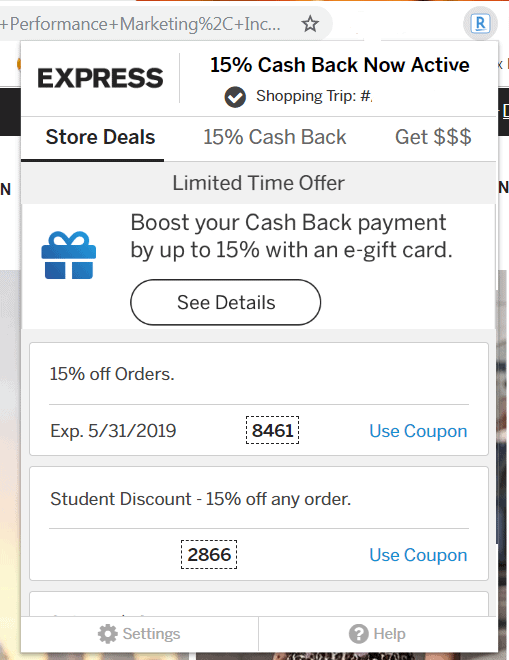On the Express store website, a prominent pop-up window dominates the screen, partially obscuring the website's main interface. The frame of the website is faintly visible around the edges. At the top of the pop-up, on the left-hand side, is the Express logo.

The central message of the pop-up, in bold black lettering, announces that "15% Cash Back Now Active." Below this, a gray box with a white check mark contains the phrase "Shopping Number."

The pop-up is divided into sections for ease of navigation:

1. **Store Deals** - Highlighted in black and underlined, indicating it is the current selection.
2. **15% Cash Back** - Grayed out, not currently selected.
3. **Get Money ($$$)** - Also grayed out and not active.

Centered below these sections, the text "Limited Time Offer" grabs attention.

Further down, the pop-up features another rectangle containing the image of a present, accompanied by the offer: "Boost your cashback payment by up to 15% off with an e-gift card." Below the image, a prominent oval button, labeled "See Details," invites users to learn more.

At the bottom of the pop-up, a final rectangle displays the offer details: "15% Off Orders." The offer expires on 5/31/2019. A hyperlink labeled "Use Coupon" is provided, with a coupon code "8461" enclosed in a dotted box for easy reference.